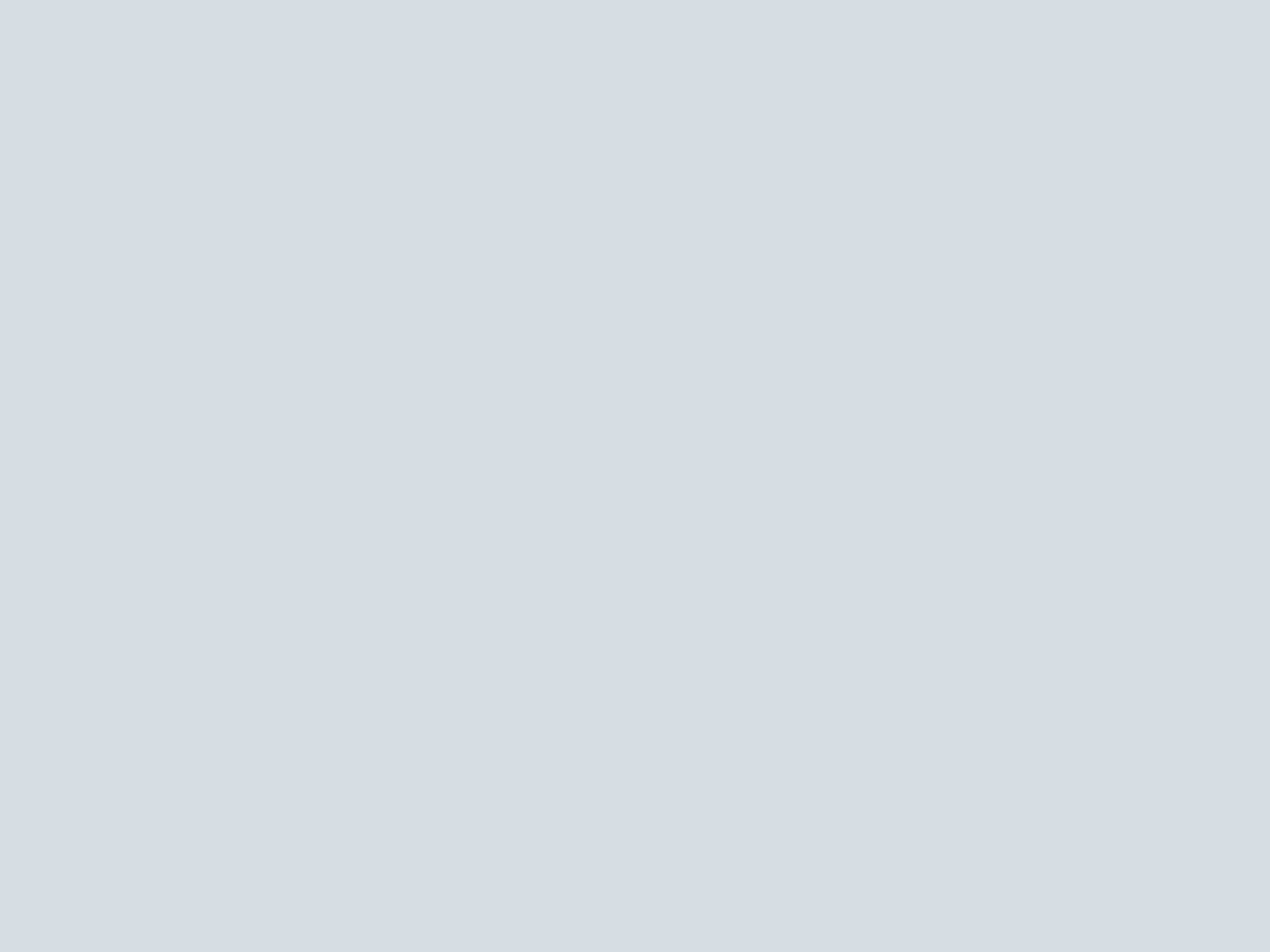This image features a large, empty square with a uniform battleship gray color, set against a stark white background. The square is meticulously even on all sides, clearly defining it as a geometric square. Its size appears to be at least 10 inches per side, creating a significant visual presence on the white canvas. The absence of any content within the square opens up imaginative possibilities about its intended purpose or what it could potentially contain. The simplicity of the gray box contrasts sharply with the brightness of the background, suggesting it could be a section of a computer screen or a snapshot from a catalog page, showcasing a blank space reserved for future content. The overall minimalist design and the precise coloring capture attention, inviting contemplation and interpretation.